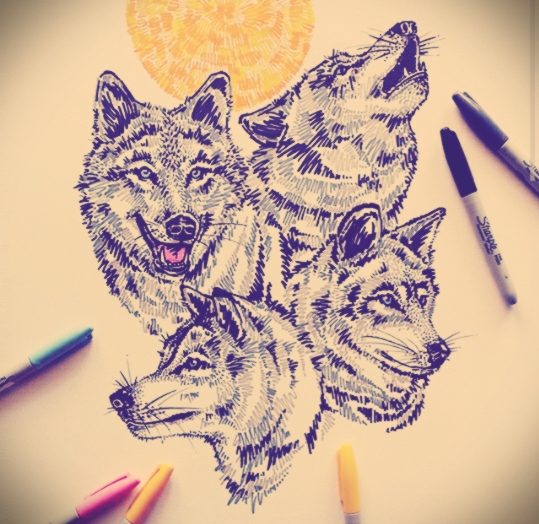The image showcases a detailed drawing on white paper featuring a vibrant sun and four intricately illustrated wolf heads, each expressing different characteristics. The sun, drawn in a unique style with lengthwise yellow and orange lines forming a circle, crowns the composition. Below the sun, the four wolves are arranged, each portrayed with meticulous attention to detail, emphasizing fur texture and whiskers.

The wolf on the far left is depicted in black and white with strikingly light blue eyes, its mouth open to reveal a pink tongue. To its right, another wolf is shown howling upwards, likely at the moon, its head tilted back. The bottom left wolf presents a side profile looking to the right, its whiskers prominently featured. The final wolf, towards the upper corner, looks straight ahead but slightly to the side, adding to the dynamic presentation of the heads.

Scattered around the top of the paper are various markers: a black Sharpie, two shades of yellow, pink, and blue, suggesting these were the tools used for this detailed artwork. This intricate depiction of the sun and wolves, with emphasis on the wolves' wet noses, sharp whiskers, and expressive eyes, showcases the artist's skill in capturing detailed textures and lifelike features.